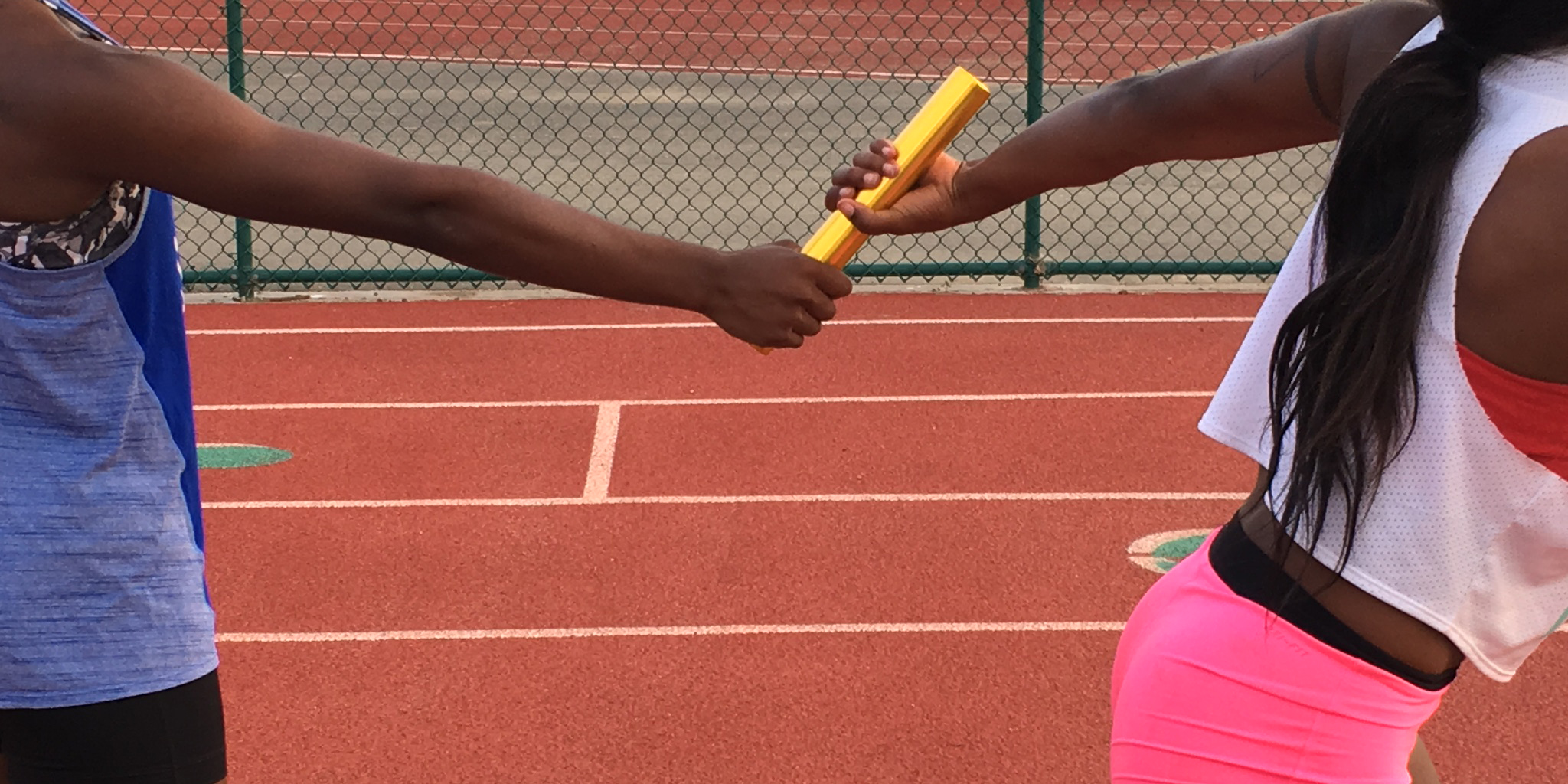The photograph captures an intense moment during a relay race featuring two athletic Black women in mid-handoff. The scene focuses on the critical exchange of the golden baton, occurring on an orange running track marked with lines. The background includes a green chain-link fence, helping to frame the action. The runner on the left side of the image, partially visible from her thigh to shoulder, wears a blue tank top, black shorts, and a sports bra. Her right arm extends forward, gripping the base of the baton. The runner on the right, mirrored in visibility from shoulder blade to upper thigh, dons neon pink shorts and a white mesh tank top with a sports bra underneath, her hair secured in a ponytail. She reaches back with her left hand to grasp the baton firmly towards the top, poised to continue the race without losing momentum. Both women are captured at the precise moment they simultaneously hold the baton, epitomizing the coordination and timing essential in a relay competition.